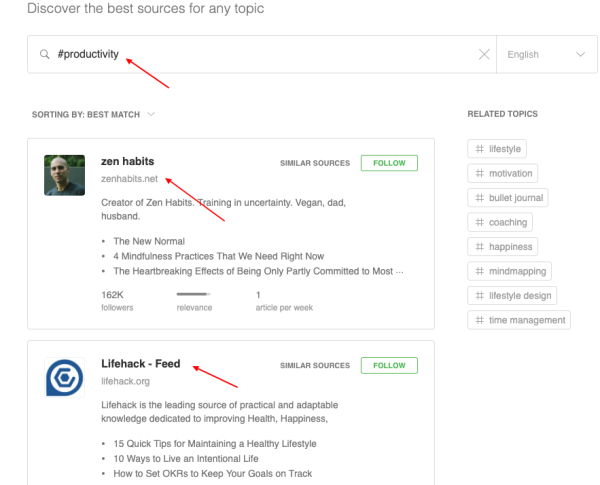This image displays a screenshot set against a white background. At the top, there is a bold heading that reads, "Discover the Best Sources for Any Topic." Below this heading is a search bar with a magnifying glass icon, accompanied by the hashtag "#PounceOnProductivity." A prominent red arrow points to the word "productivity."

On the right side of the screenshot, there is a profile section for "Zen Habits," which includes the creator's profile picture. Key details about this profile include descriptors such as "creator of Zen Habits, training in uncertainty, vegan dad, husband." Additionally, the profile highlights several articles, namely "The New Normal: Four Mindfulness Practices that We Need Right Now" and "The Heartbreaking Effects of Being Only Partly Committed to Most." The profile displays a count of 162k followers and a green 'Follow' button.

A second red arrow points to the text "zenhabits.net," the official Zen Habits website. 

In the middle section of the screenshot, another profile titled "Lifehack Feed" is highlighted with a thumbnail featuring a blue circular icon. This profile is described as "Lifehack is the leading source of practical and adaptable knowledge dedicated to improving health, happiness." Similar to the Zen Habits section, this profile also includes a green 'Follow' button.

The image effectively organizes key information and directs attention using red arrows, while consistently featuring green 'Follow' buttons next to highlighted profiles.